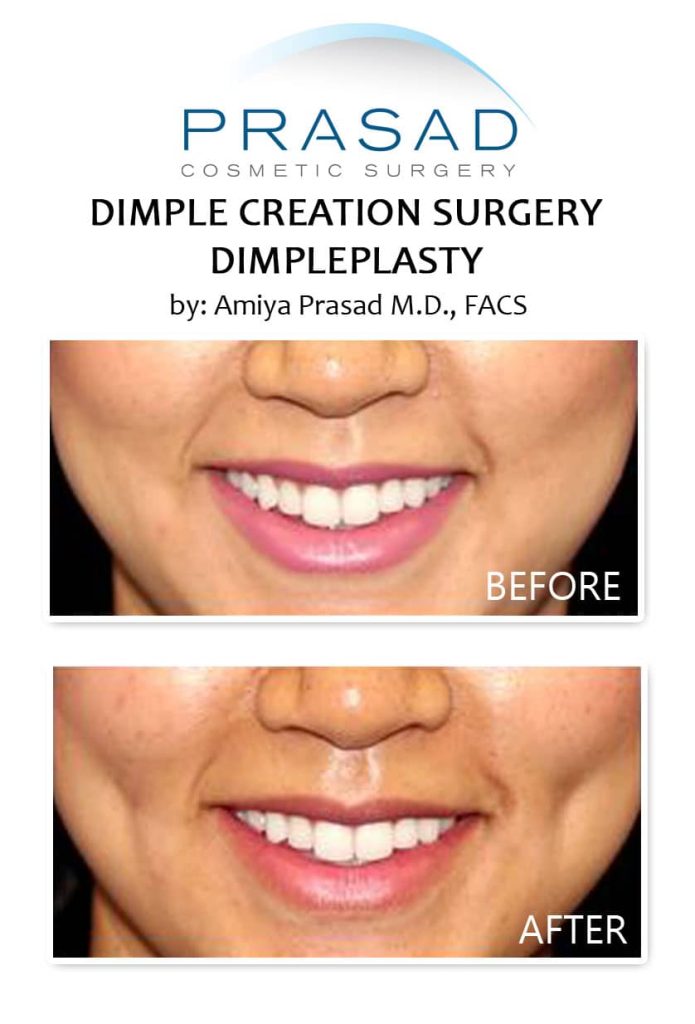**Before and After Transformation: Dimple Creation Surgery**

Top section features the name "Prasad" in a blue hue, followed by "cosmetic surgery" in gray. In black text, the caption reads "dimple creation surgery, dimpleplasty." The surgical work, attributed to Dr. Amaya Prasad, M.D., F.A.C.S., showcases a portfolio item intended for the website.

The image is divided into two rectangles: the first, labeled "before" in the top right corner, shows the patient's initial state. The adjacent rectangle, marked "after," displays a subtle yet noticeable enhancement of dimples post-surgery. The side-by-side comparison highlights the successful results of the cosmetic procedure, despite the minimal variations at first glance.